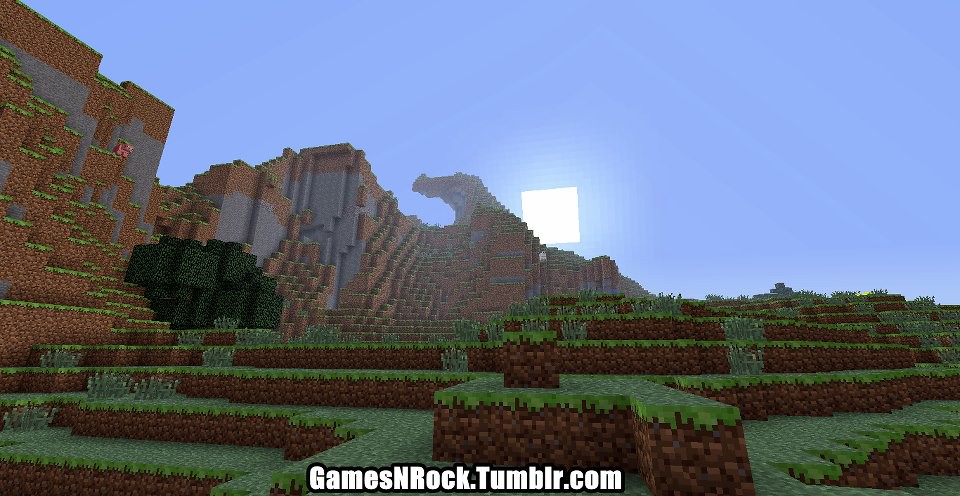This digital image showcases a distinctly pixelated, blocky landscape that appears to be constructed entirely of square blocks, evoking a video game aesthetic. The ground is composed of brown square blocks, resembling rocks or dirt, with a layer of lush green grass atop them. These grassy dirt blocks ascend in a stair-like fashion from the bottom left towards the top right, creating a terraced hillside that reaches halfway up the image. Scattered across the grassy blocks are various small green plants, adding to the detail. The sky overhead is a clear blue, punctuated by a solitary white square at the center of the scene. On the left side of the image, a towering blocky mountain, also brown, adds to the rugged terrain. Between the two brown mountains, a dark, shadowed area of blocks creates a striking contrast, further defining the landscape's depth and dimension.